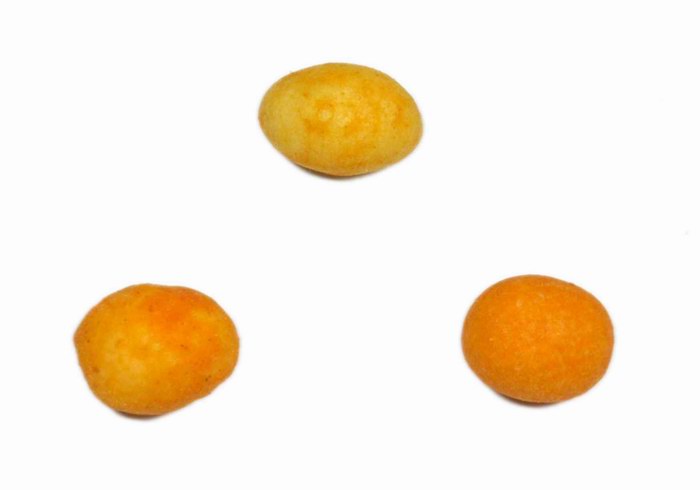In this photo with a white background, three spherical objects are arranged in a triangular formation. The top object resembles a Yukon potato with a yellow hue and orange markings, casting a faint shadow below it. The bottom left object looks like an orange ball of cheese with yellowish spots, resembling fried food with a slightly rough texture. The bottom right object appears similar to a tangerine with a thick orange peel, suggesting a firm and textured surface. Despite the image being somewhat fuzzy and lacking distinct details, these objects appear to be food items, possibly biscuits or fried treats, characterized by their circular shape and smooth surfaces.